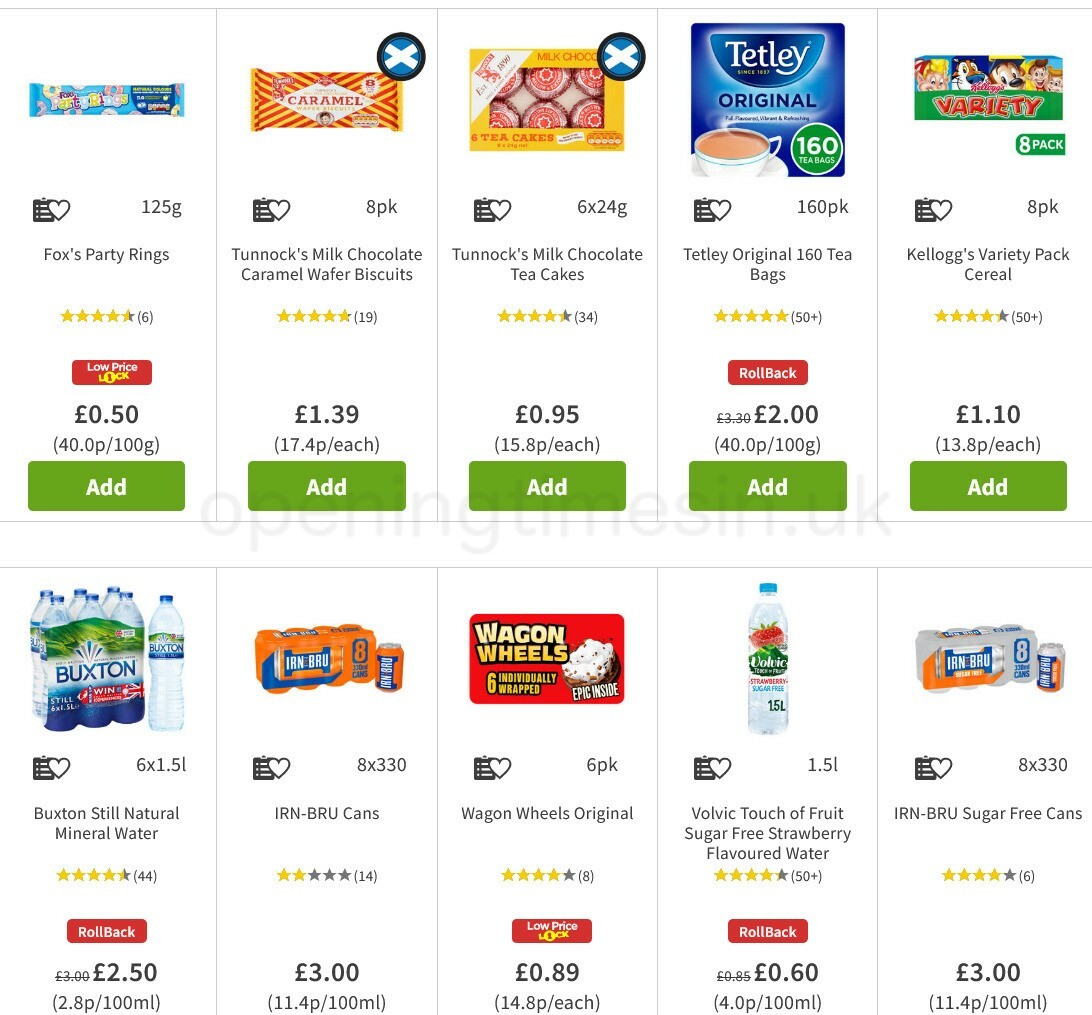Here's a detailed and cleaned-up caption for the image:

---

This is a vibrant screenshot captured from an online store displaying an assortment of food and beverage items organized neatly in two rows. 

In the first row:
1. *Fox's Party Rings*: A colorful pack of party-themed biscuits priced at 50 pence. Below this item, a green button with white lettering says "Add" to enable easy addition to the cart.
2. *Caramel 8-Pack*: A set of Tonics Milk Chocolate Caramel Wafer Biscuits, attractively priced at £1.39.
3. *Tonics Milk Chocolate Tea Cakes*: Priced at 95 pence (£0.95), these delightful treats are perfect for tea time.
4. *Tatley Original Tea Bags*: A pack of 160 tea bags, originally priced at £3.30 but now available for £2.
5. *Cal Love's Variety Pack Cereal*: An eight-pack assortment of cereals costing £1.10.

In the second row:
1. *Buxton Steel Natural Mineral Water*: Bottles of mineral water priced at £2.50.
2. *IRN-BRU Cans*: A popular soda with distinctive orange packaging, available at £3.
3. *Wagon Wheels Original*: Individually wrapped cakes in a six-pack, priced at 89 pence (£0.89).
4. *Volvic Touch of Fruit Sugar-Free Strawberry Flavored Water*: On sale for 60 pence (£0.60), featuring a rollback sign to indicate the discount.
5. *IRN-BRU Sugar-Free Cans*: A sugar-free version of the beloved soda also priced at £3.

Each item features a green "Add" button beneath it for easy shopping convenience.